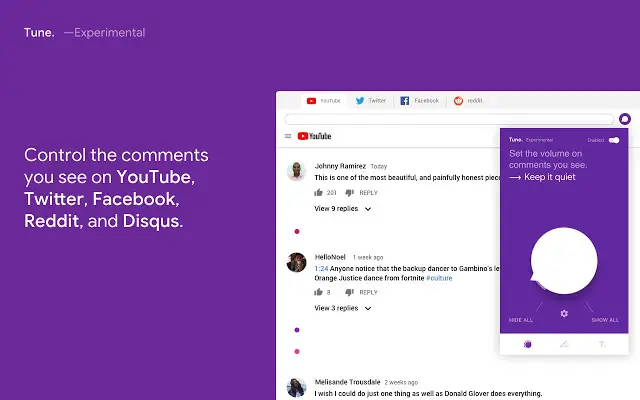This advertisement highlights a feature called "Tune," labeled as "experimental", that enables users to control the comments they see across various social media platforms. The top-left corner of the image features the text "TUNE." in bold white, followed by "experimental" in a lighter white font. A vivid purple background emphasizes the main advertising message, which is displayed in white text: "CONTROL THE COMMENTS YOU SEE ON YOUTUBE, TWITTER, FACEBOOK, REDDIT, AND DISQUS."

In the bottom right corner, an illustration of a web browser is showcased, displaying four open tabs: YouTube, Twitter, Facebook, and Reddit. The content within the active YouTube tab reveals several comments, including "Johnny Romeres: This is one of the most beautiful and painfully honest..." and another comment referencing a backup dancer from Fortnite, followed by a message expressing admiration for Donald Glover. Additionally, three dots indicate where comments have likely been filtered out by Tune's service. 

To the right, an interactive feature of Tune is described: "SET THE VOLUME ON COMMENTS YOU SEE, KEEP QUIET." A white knob is depicted, suggesting that users can rotate it to increase or decrease the number or type of comments they receive. The advertisement effectively illustrates Tune's capability to manage social media interactions by filtering out unwanted content.